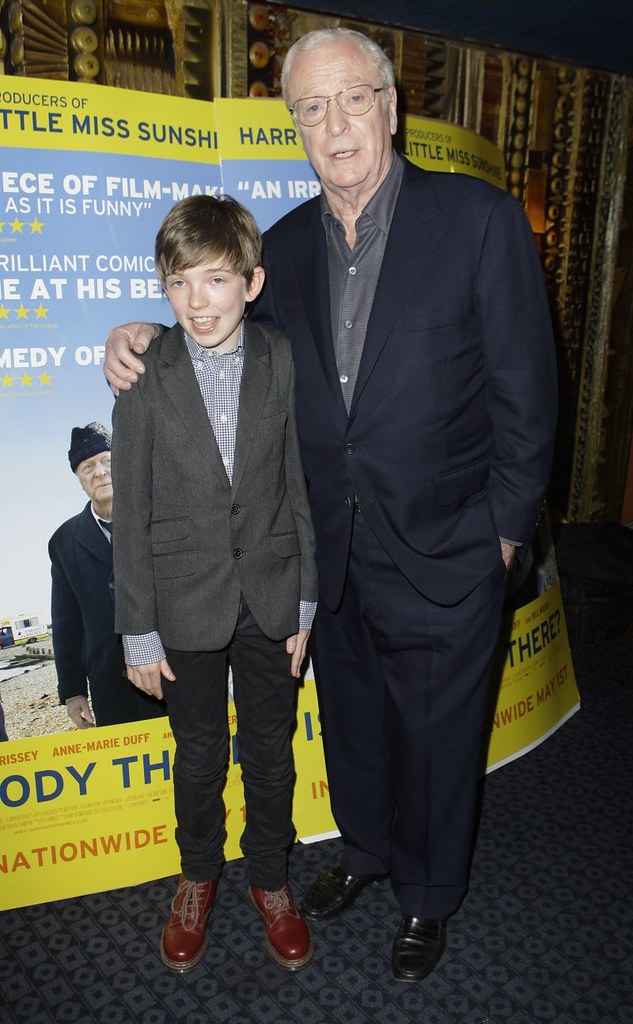In this indoor photo, an older man and a young boy are standing on a gray and black carpet, likely at a movie premiere event. The backdrop is a large advertisement or billboard for the movie "Little Miss Sunshine," featuring partially visible text such as "producers of Little Miss Sunshine" and phrases like "filmmaking brilliant comic." The man, dressed in a dark blue suit with a gray shirt and black shoes, has gray, thinning hair and wears glasses. He stands to the right of the boy, with his right arm affectionately draped around the boy's shoulders. The boy, around 10 years old, wears a gray sports jacket over a blue button-down shirt, dark blue pants, and brown shoes. He has light brown hair and a big smile on his face. Behind them, the poster displays hues of yellow, blue, white, and brown, and above it, a hint of a gold-colored wall is visible.